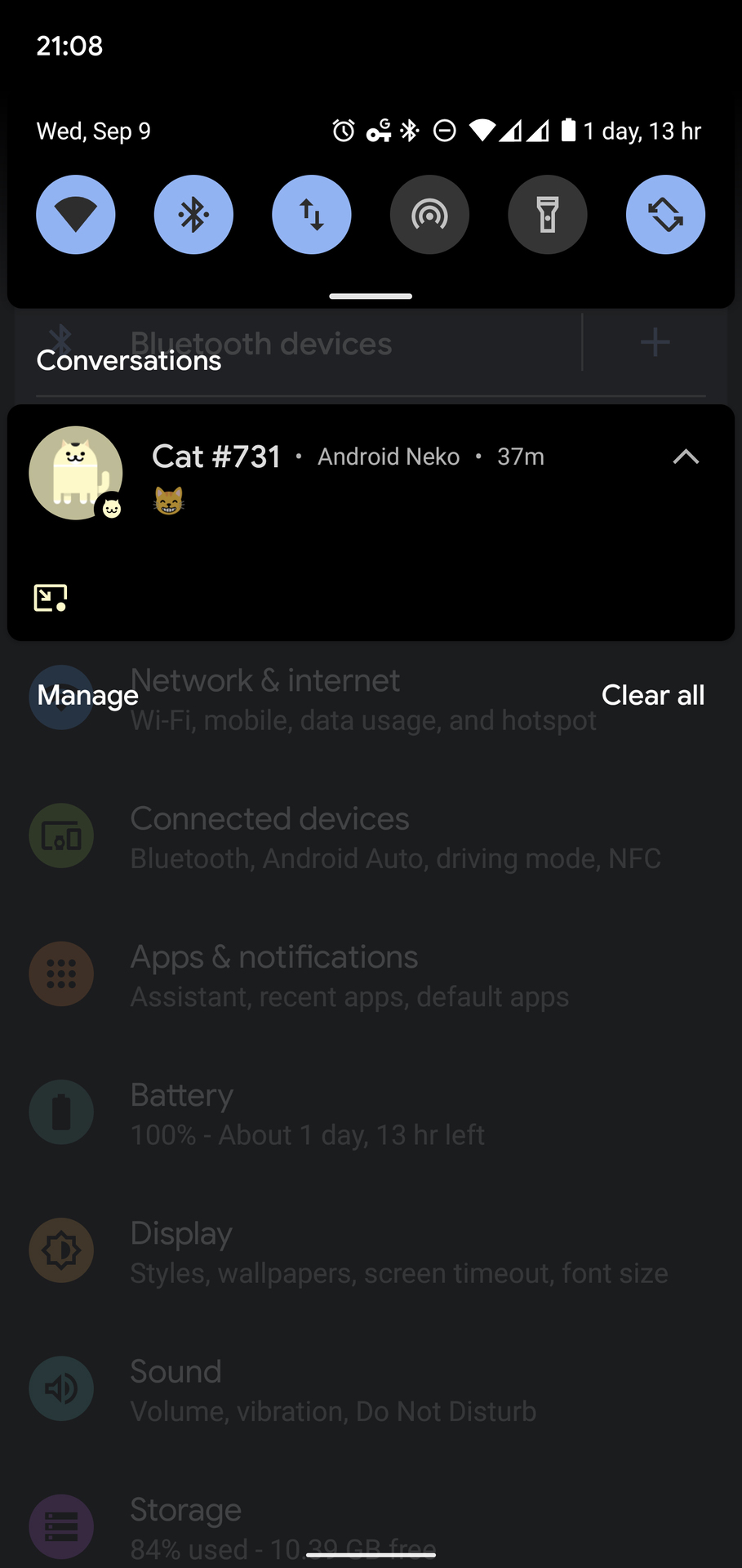A smartphone screenshot displaying various system information and status indicators. At the top, the screen shows the time in military format as "21:00" and the date as "Wed, Sep 9." There are several icons indicating system statuses, including an alarm clock, a key, Bluetooth, a minus sign inside a circle, Wi-Fi strength, battery level, and a battery with an estimated one day and 13 hours of charge left.

Below these indicators, there are four highlighted icons representing active features: Wi-Fi, Bluetooth, Exchange, and a circular synchronization symbol. Next, under a section titled "Conversations," the screen displays "Cat #731 - Android Nico" indicating a conversation that lasted 37 minutes, accompanied by a circular icon featuring a white cat and an orange emoji with bared teeth.

There is a smaller section below the conversation details including a diagonal bar and options to "Manage" (on the left side) and "Clear All" (on the right side). The options and the text are white. 

Towards the bottom, there are categories like "Network & Internet" which shows a blue circle, and another green circle suggesting connected devices including Bluetooth and others. Other categories listed include "Notifications," "Battery," "Display," "Sound," and "Storage."

The entire screen has a black background, emphasizing the icons and text in bright colors for contrast.